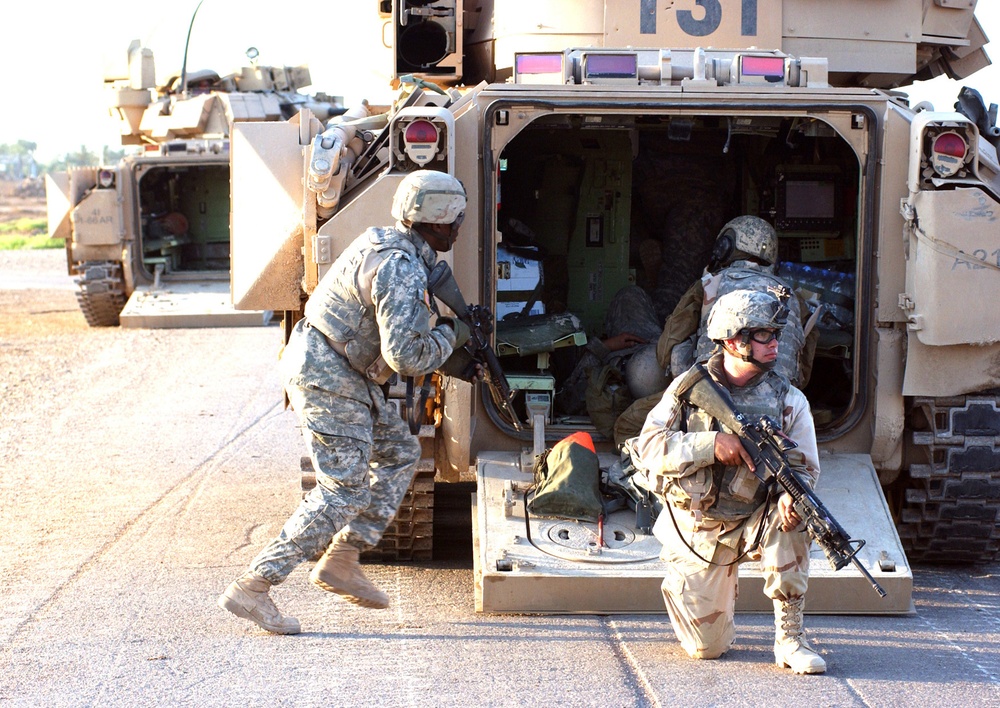In this detailed image, military soldiers are engaged in a medical evacuation training exercise surrounding two tanks, one on the left and one on the right. The prominent tank on the right is open, revealing an injured soldier lying inside while being attended to by a medic. The medic kneels with his left knee raised, tending to the injured man who has his left arm draped over his chest. Another soldier is entering the tank, standing on both feet and wielding a rifle, while a third soldier, also carrying a rifle, kneels on one knee near the tank facing the camera but looking off to the side, appearing vigilant. All soldiers are in full camouflage gear, complete with helmets and rifles. The scene is brightly lit, indicating daytime, and to the left in the background, the second tank waits, suggesting readiness for further action.